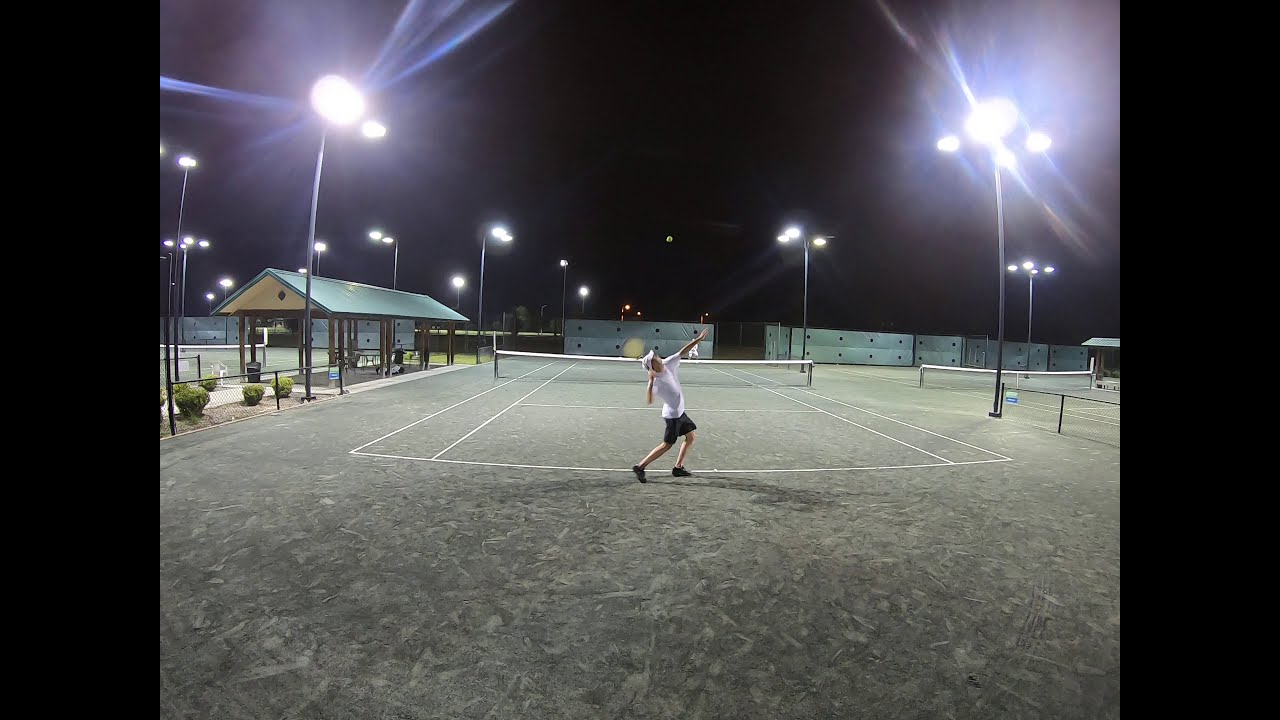On a brightly lit tennis court at night, a player in a white T-shirt, black shorts, black shoes, and a white cap is poised to serve the ball, which is captured mid-air above him. The grey court with white outlines is illuminated by tall poles with bright lights. The net, featuring a white trim, divides the court. In the background, another player stands at a distance, barely noticeable in the shadows. To the left side of the image, a booth with a circular green roof and wooden pillars stands, accompanying some benches under the shaded area. The sky is pitch black, emphasizing the vivid lighting on the court, making the scene distinctly clear and focused.